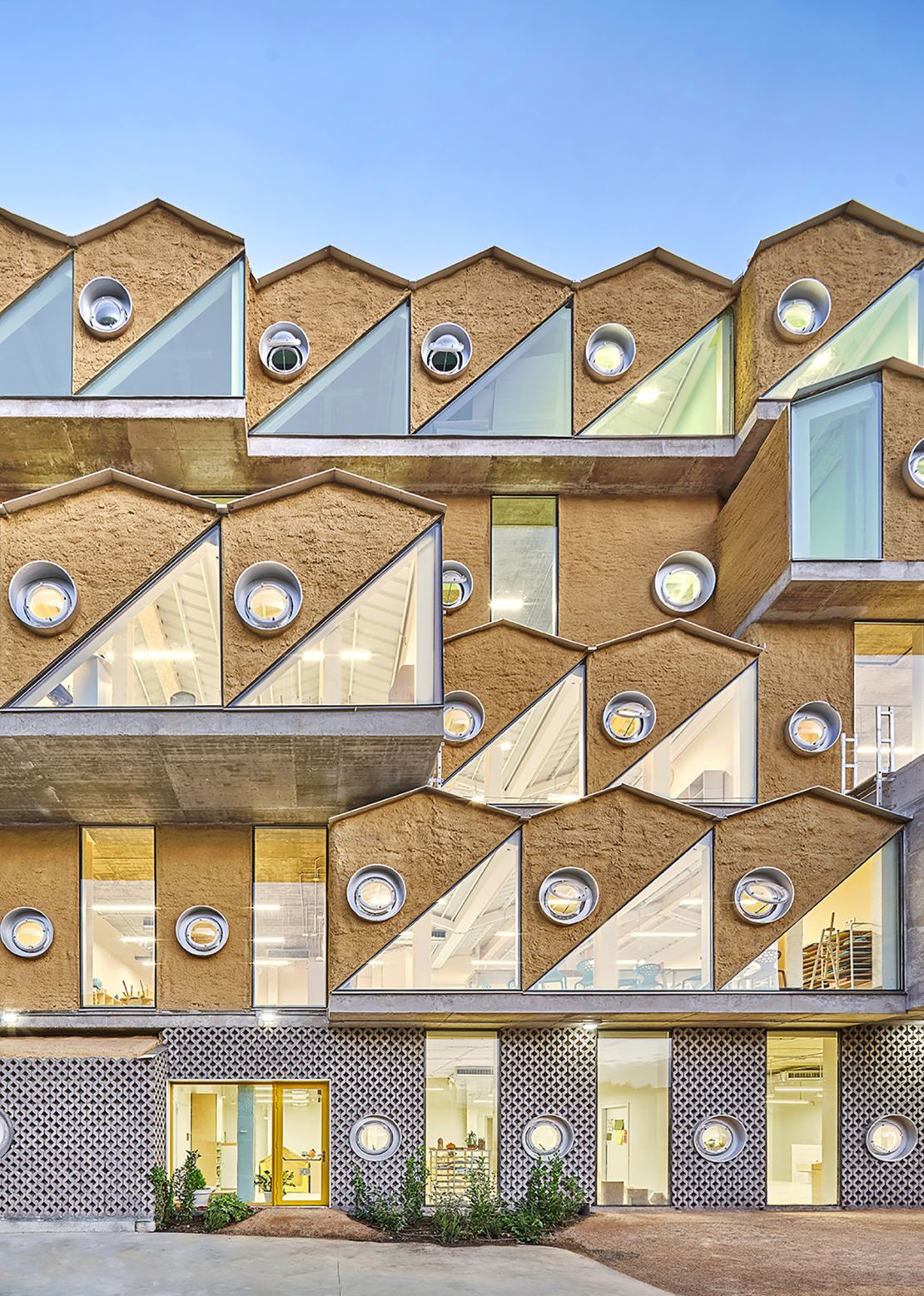The image portrays a modern, uniquely structured building with five unevenly stacked floors, possibly a 3D rendition. The bottom floor features a crosshatched silver façade accented by tall, rectangular floor-to-ceiling windows, accompanied by smaller round porthole windows interspersed between them. A patio door is discernible on the left-hand side, flanked by a couple of bushes, with the ground transitioning from dirt on the right to asphalt on the left.

Above this level, the design shifts dramatically. The next three floors consist of these peculiar pentagon-like units. Each unit displays a distinctive pattern with half of the façade in a stucco tan or brown hue, encompassing small round windows. The bottom half of each pentagon is adorned with triangular, possibly grayish-clear windows. These elements create a sense of depth as alternating sections jut out away from the building while others remain recessed, forming overhangs.

The final floor follows a similar pentagon motif but is more pronounced, with the side sections jutting further out and the central section recessed. All floors exhibit a blend of rectangular and round windows, contributing to the overall eclectic architectural style. The backdrop features a clear, light blue sky, adding a serene contrast to the building's modern and somewhat abstract design.